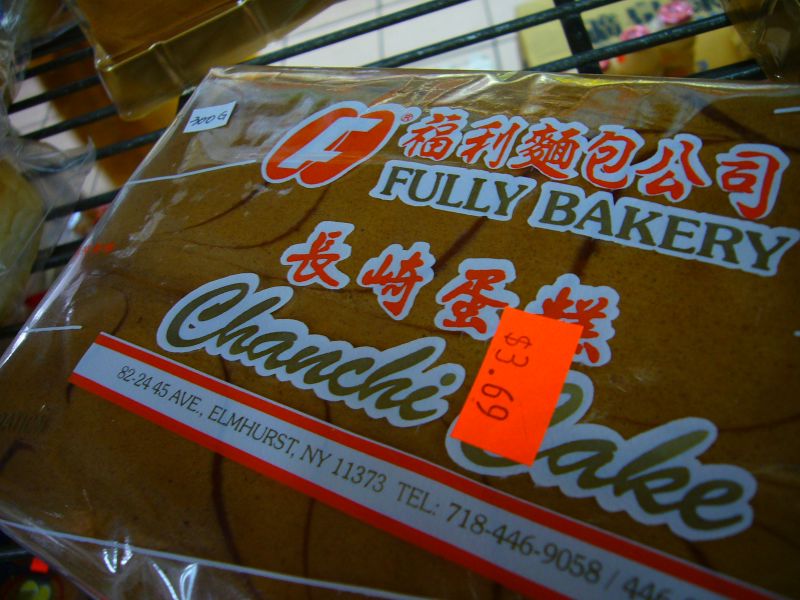This close-up photograph captures a packaged item, possibly a cake or a loaf of bread, encased in clear plastic cellophane. The packaging is adorned with various texts and symbols. At the top of the package, there are red Chinese characters, followed by the words "FULLY BAKERY" in green, prominently outlined in white. Next to them, additional Chinese characters are displayed in red, also outlined in white. Beneath this, there is green text reading "CHANSHEE BAKE," also outlined in white. A red price tag marked $3.69 is partially placed over the letter B in "BAKE." Below this, a white bar bordered in red contains a green address: "82-24 45th Avenue, Elmhurst, New York, 11373," along with the telephone number "718-446-9058." The image appears to be taken indoors, potentially in a Chinese supermarket, with black wire shelving and other indistinct items visible in the background.